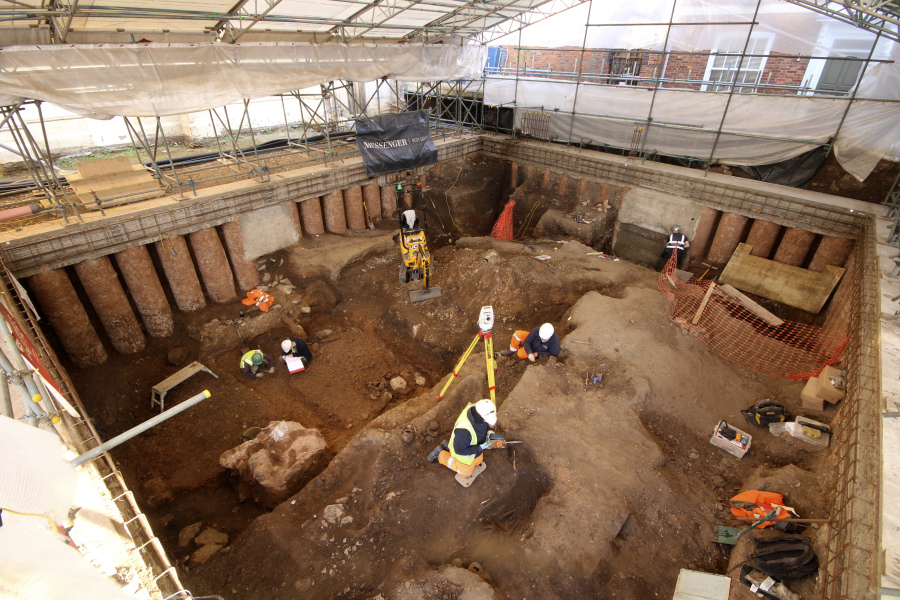The photograph depicts a bustling excavation site, meticulously structured in a square formation and shielded by scaffolding and plastic coverings to protect against the elements. The site, approximately 15-20 feet deep from ground level, shows signs of significant activity as four to five workers meticulously dig and measure within. At the center of the activity are remnants of what appear to be ancient Greek columns, hinting at the historical importance of the dig. Amidst the mounds of excavated dirt, various surveying equipment and construction tools are scattered, indicating ongoing measurements and evaluations.

The scaffolding structure not only marks the perimeter but also provides a vantage point from where one can see both the excavation site and an adjacent building to the right. The frame of the site, already established with some brickwork, holds an intense focus with men engaged in various tasks: some are perched on dirt mounds using digital leveling tools while others analyze the ground or consult open books, suggesting detailed record-keeping and planning.

Tools and a machine designed for digging are visible, emphasizing the site's readiness for extensive excavation work. The overall scene portrays a well-organized construction environment where history, architecture, and modern techniques converge in a symphony of purpose and progress.